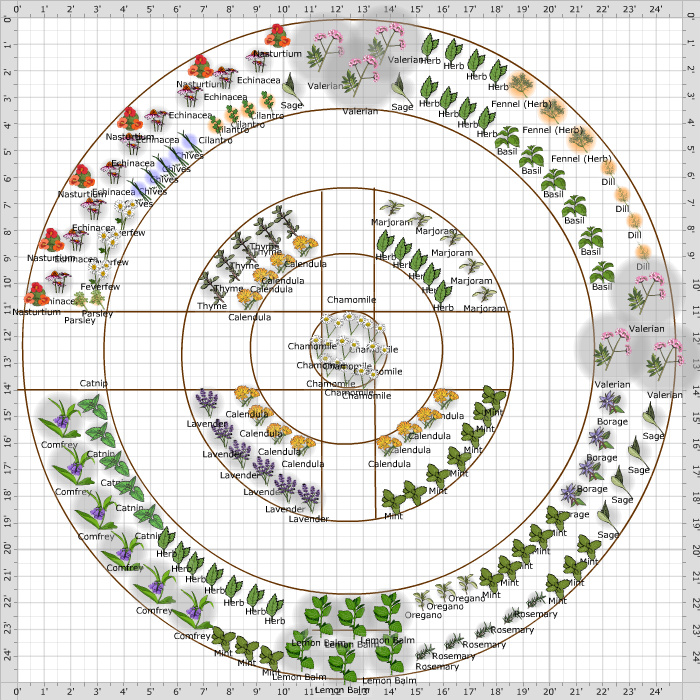This image is an intricate, line-art illustration of an herb garden superimposed on a 25-inch square grid background. The grid lines are marked from 0 to 24 inches along all four sides. At the center is the innermost circle, spanning 2 inches, labeled with chamomile and adorned with small chamomile flowers. Surrounding it are three additional concentric circles creating distinct sections for various herbs. 

A cross-shaped walkway intersects the second ring, dividing it into four labeled quadrants: marjoram and thyme in the upper left, marjoram and herb in the upper right, calendula and mint in the bottom right, and lavender and calendula in the bottom left. Each quadrant features simplistic line drawings of the corresponding herbs.

The third circle, mostly solid except for a left walkway segment, contains various herbs including nasturtiums, echinacea, cilantro, and sage. Other sections within this ring house herbs like basil, dill, valerian, catnip, comfrey, oregano, lemon balm, fennel, and borage. The outermost circle completes this meticulously organized garden illustration, offering a clear, visual layout of an abundant and diverse herb garden. The labels are cleanly typed, enhancing the clarity and instructional nature of the illustration.